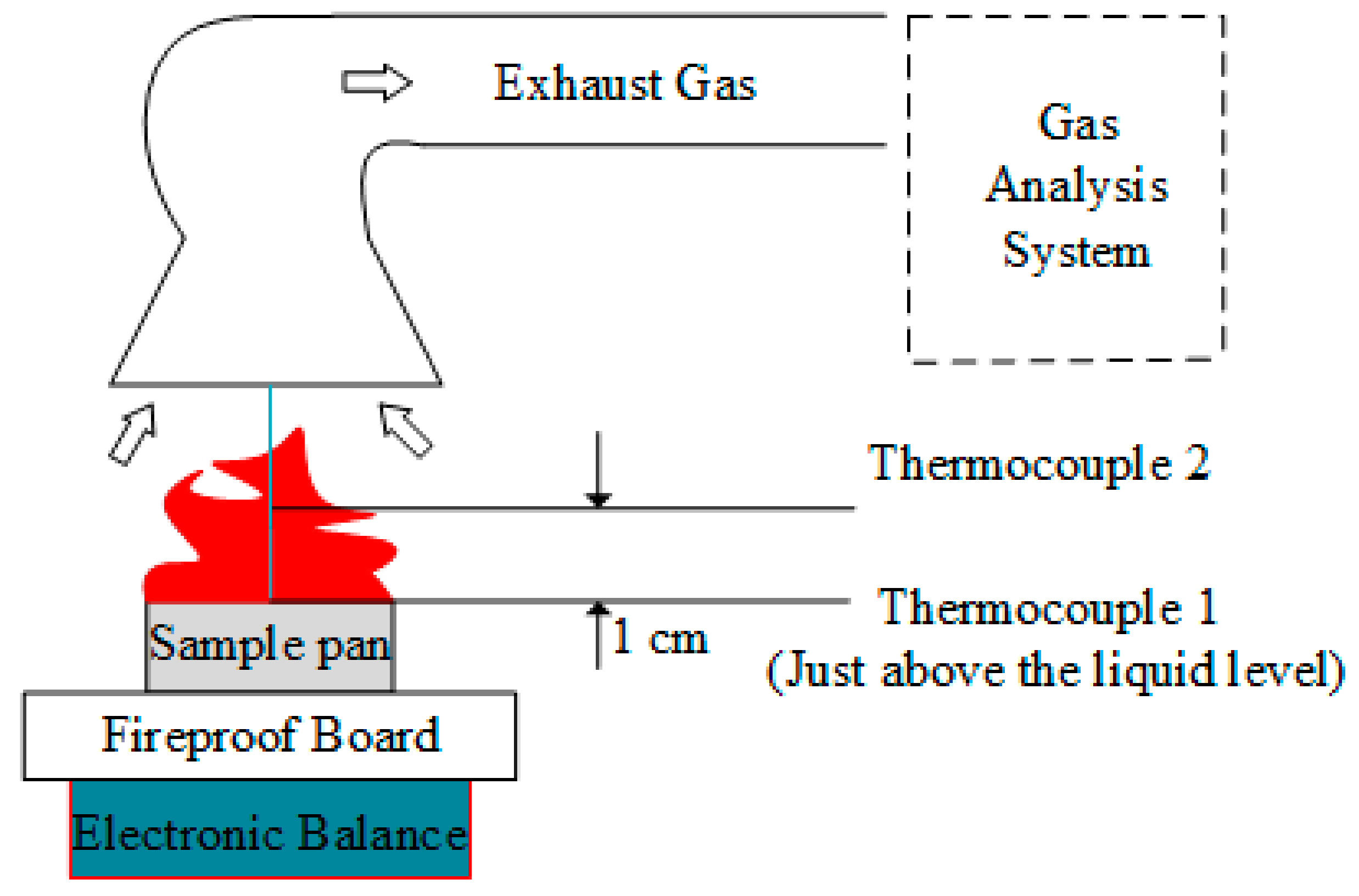This detailed diagram, set against a white background, illustrates the flow of exhaust gas through a system, serving as an educational example. At the bottom of the schematic, three interconnected levels are distinctly colored and labeled: a blue layer marked "Electronic Balance," a white "Fireproof Board," and a gray "Sample Pan" where red-colored flames indicate combustion. From these flames, arrows trace the movement of exhaust gas up into a funnel-shaped hood and onwards into a "Gas Analysis System" housed within a square box, depicted with dashed lines. The diagram includes two thermocouples immersed in the flames for heat sensing; "Thermocouple 1" is positioned just above the liquid level with an indication of 1 centimeter, while "Thermocouple 2" is placed higher up within the flames, each highlighted by directional arrows. This schematic underscores the intricate measurement and analysis of combustion gases.